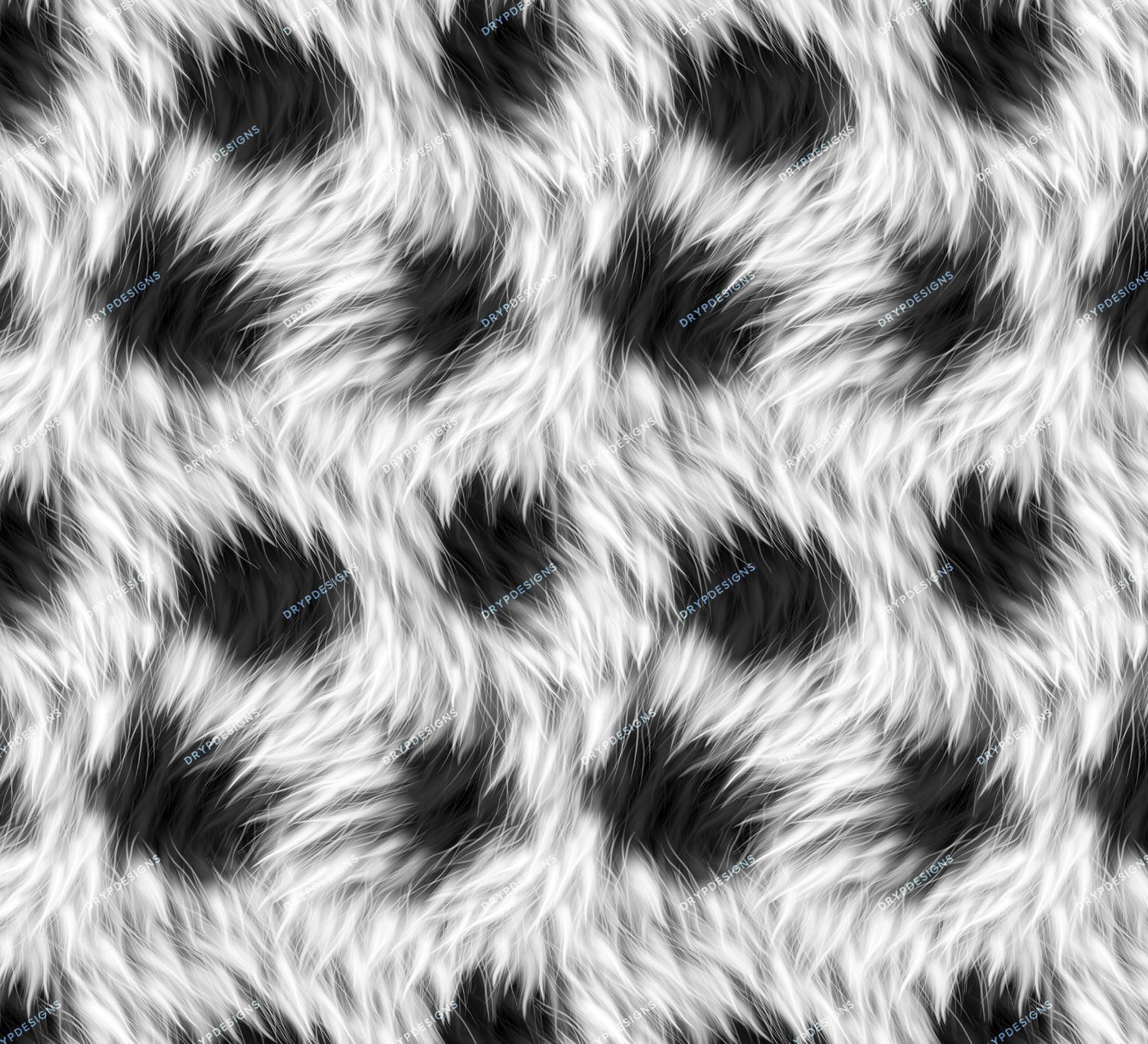A close-up digital artwork featuring a mesmerizing white and black fur-like texture against a dark backdrop. The intricate pattern is populated by black round circles, spaced in a regular yet staggered arrangement, creating an artistic sense of order. Each black circle is adorned with the text "DRYP DESIGNS" in bold, white, all-uppercase diagonal letters, forming an unbroken sequence across the canvas. The image contains approximately eight diagonal lines of this text, distributed evenly from top to bottom, imparting an organized, yet dynamically staggered feel. The ethereal wisps of white mimic the look of fur, blending seamlessly into the circular black elements, while the overall monochromatic color scheme accentuates the striking contrast between the elements. The entire composition creates a surreal, almost hypnotic design that is both structured and fluid.